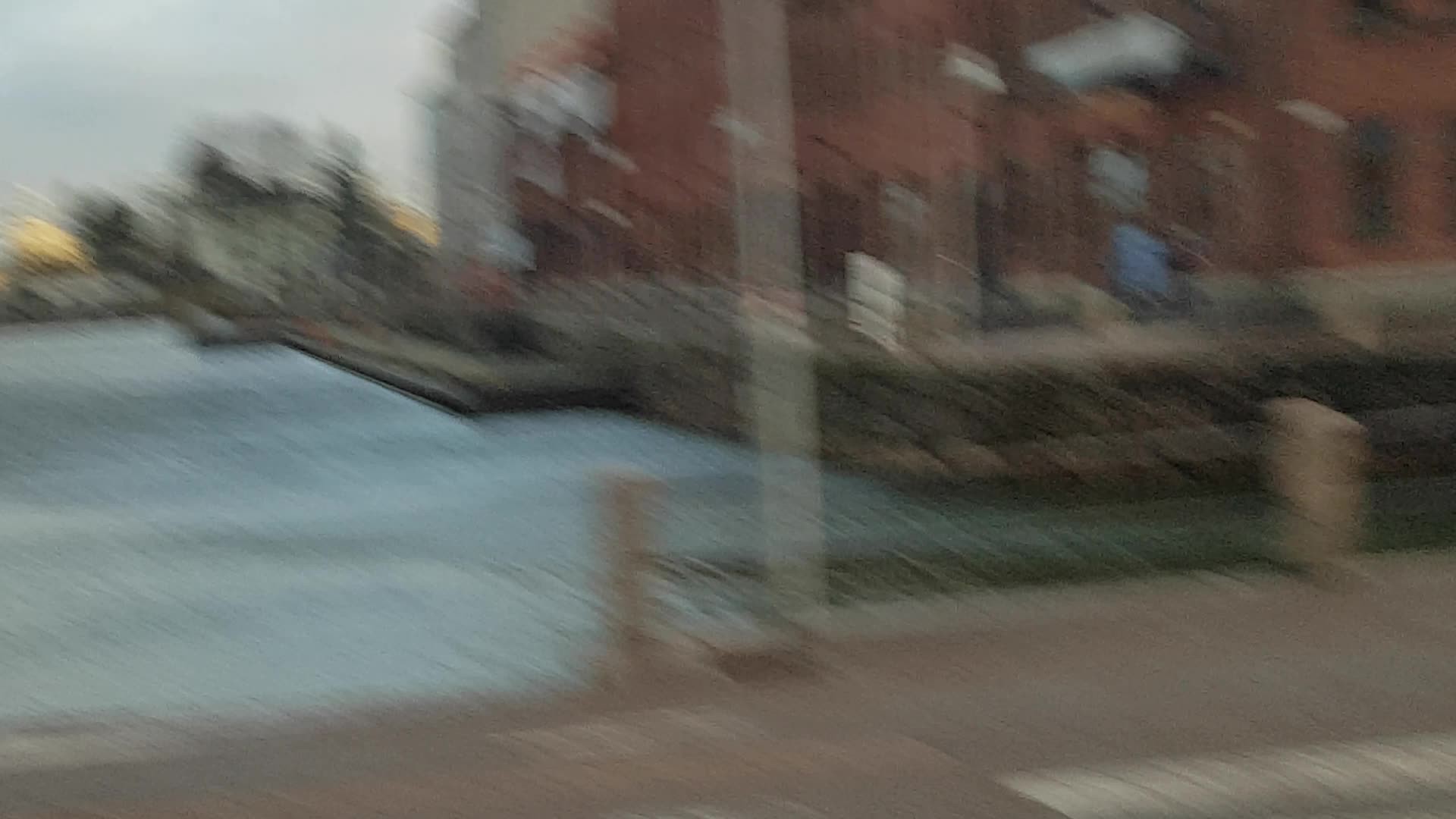In this horizontally-oriented, rectangular image, we observe an extremely blurry and low-resolution photograph showcasing a section of a walkway. The walkway extends diagonally from the lower left to slightly higher on the right. Alongside this walkway, there is either a railing or a long, narrow bench. The walkway is brown, the bench seat is dark, and the sides of the bench are a lighter tan.

Beyond this walkway, there is a red brick structure with unclear details regarding windows or doors. However, there are some darker areas on what appears to be the first floor. Light is shining from above, casting little glints along the base of the red brick building, suggesting reflections or minor illuminations. Additionally, in the lower right corner, there is a shadow, possibly cast by sunlight.

In the upper left corner, a bit of light blue sky is visible, adding to the overall serene, albeit blurry, atmosphere of the photograph.